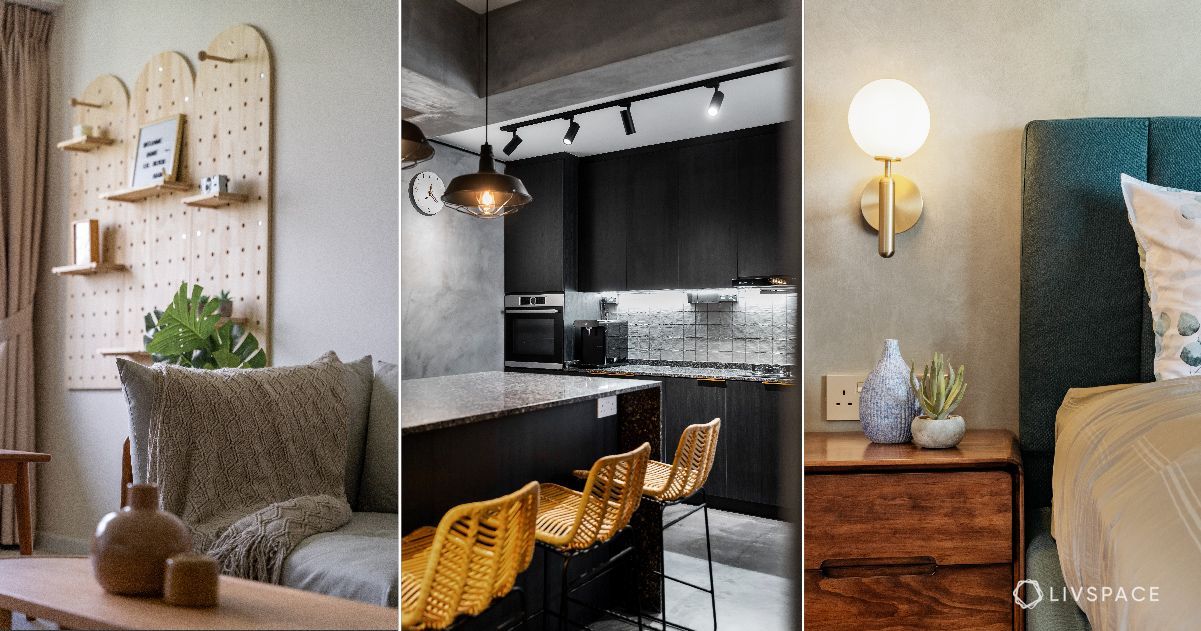The tripartite image showcases different rooms of a highly stylized living space. The image on the left depicts a tan-themed living room featuring a couch with a cover, a pegboard-style art installation adorned with various items like a camera and a box, as well as floating shelves and a poster. The coffee table in front of the couch is adorned with a vase or pottery, and the room has an overall warm, monochromatic tan decor. 

The middle image presents a sleek, modern kitchen characterized by black cupboards and appliances, complemented by gray walls and a silver backsplash. The centerpiece of the kitchen is a gray granite island surrounded by three brown wicker stools, with a trio of orange stools also mentioned. The kitchen also features track lighting, a yellow-hued hanging lamp, and a clock on the wall. Additional details include a wall-mounted stove and oven.

The image on the right showcases a cozy bedroom with a partial view of a blue or dark green headboard and tan sheets. The wooden bedside table is adorned with a plant and a decorative vase. The room is lit by a large wall sconce with a globe light, adding a subtle touch of elegance. Notably, a European wall plug is visible. The bottom right of the composite image displays the text "Live Space."